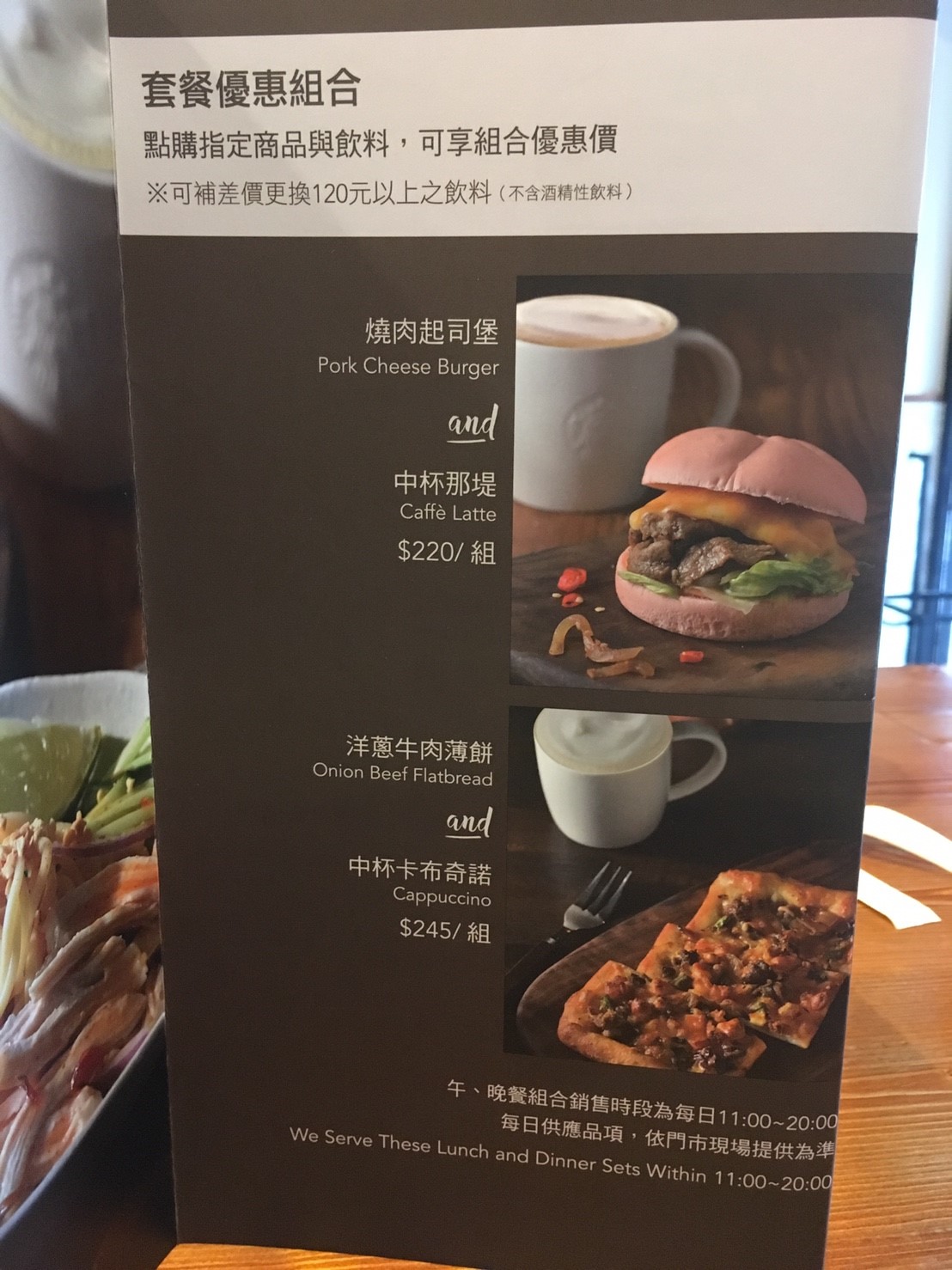This photograph showcases a specials menu prominently displayed on a rustic wooden table, whose distinct wood grain detail is evident. The table is composed of several wooden planks, adding a robust and textured aesthetic. On the right-hand side of the image, part of a window or a pole can be seen, suggesting the setting might be a cozy coffee shop or a restaurant.

The menu, styled with a sophisticated black and white theme, features a broad white stripe along the top, approximately one centimeter thick. Inside the stripe, various details are written in an Asian language, likely Japanese or Chinese. The top portion features a bold heading, followed by a subheading, and subsequent descriptive information in smaller characters.

The main black section of the menu displays two enticing photographs on the right side. The first image shows a cup of coffee paired with a pork cheeseburger topped with cheese, served on a dark plate. Below this photograph, text in both Asian characters and English reads "Pork Cheeseburger" and "Cafe Latte," along with the respective prices.

The second photograph depicts a steaming cup of what appears to be a hot drink alongside an onion beef flatbread. The accompanying text identifies the items as "Onion Beef Flatbread" and "Cappuccino," again with prices listed.

At the bottom of the menu, additional information specifies that these lunch and dinner sets are available between 11 AM and 8 PM, with the timings indicated in the Asian language.